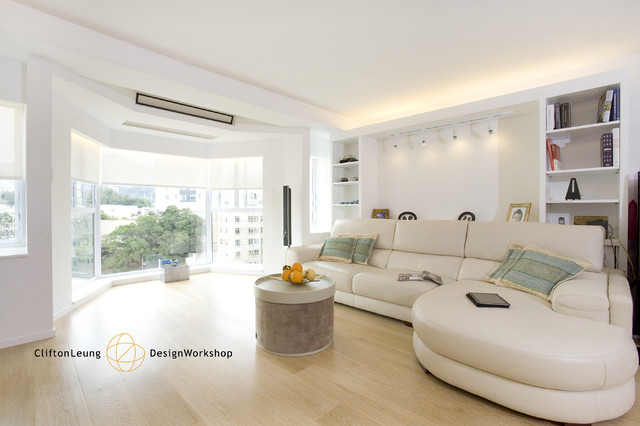This indoor photograph captures a luxurious, high-end living space with a sophisticated design. Prominently featured in the center of the room is a small, round coffee table adorned with a bowl containing several perfectly spherical oranges. To the left, an open window offers a scenic view of a park with leafy trees growing next to tall buildings, adding a touch of nature to the urban landscape. To the right, an elegant white sofa with a sectional extension is accompanied by a series of four matching throw pillows in varying shades of green and light cream accents. Additionally, a black iPad rests on the sofa, suggesting a blend of modern technology and comfort.

Behind the sofa, there is a set of bookshelves displaying an array of standing photographs and illuminated by hanging halogen lights, creating a warm, inviting ambiance. Recessed lighting further enhances the room's aesthetic with a soothing yellow glow. In the bottom left corner of the photograph, the text "Clifton Long Design Workshop" confirms the designer's sophisticated touch. The overall setting exudes an air of exclusivity, potentially hinting at an apartment of substantial value, thanks to its thoughtful design and luxurious fixtures.